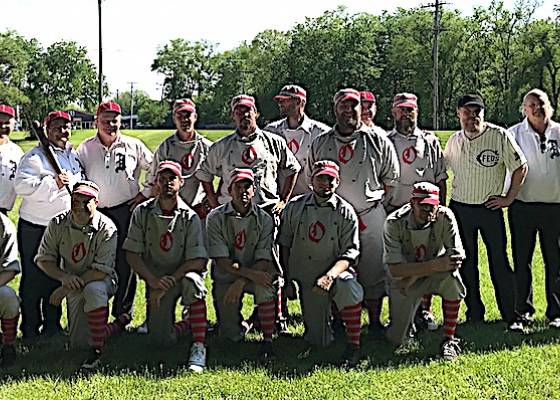This is a color photograph of a men's baseball team, likely from an earlier era, comprising about 12 to 15 members. The team is posed on a grass field, with six individuals kneeling in the front row and another row standing behind them. They are uniformly dressed in gray and red attire, featuring gray pants, gray and red striped socks, and gray shirts with six buttons resembling chef uniforms. Each shirt bears a red emblem, possibly a cursive "D," displayed prominently at the center. Their hats, which have a distinct look resembling railroad conductor caps, are gray with a single red stripe across the front and back.

The photograph also captures some variance in attire; to the far right and left of the group, individuals who appear to be coaches are dressed differently, in black slacks and white shirts, with one holding a baseball bat. The image composition is informal, with some team members looking directly at the camera while others gaze elsewhere, adding a touch of spontaneity to this nostalgic team photo.